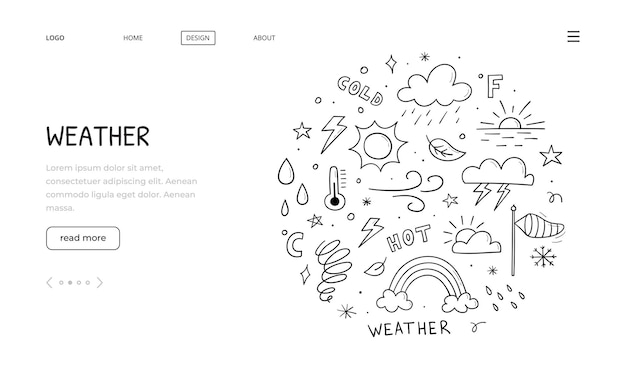The image appears to be a screenshot of a website or app, featuring a structured layout. On the top left, navigation sections are labeled as Logo, Home, Design, and About. Dominating the left side of the page, the word "WEATHER" is prominently displayed in large black capital letters. Below this header, there is placeholder text in Latin, commonly used as a dummy text in web design, known as "lorem ipsum." This section also includes a "Read More" option for extended information.

On the right-hand side, the central focus is a circular illustration depicting various weather elements in black and white. This circle is filled with numerous icons and symbols representing different weather conditions: rain clouds, a sun, swirly lines indicating wind, a cloud with lightning bolts, a rainbow, a tornado, a thermometer, lightning bolts, and images of a sunrise or sunset. Accompanying these are the words "hot," "cold," and "weather," as well as symbols such as raindrops and leaves blowing in the wind. The top right features an icon of three horizontal lines, indicating a menu for additional options. The entire layout suggests an interactive and informative weather-themed web page or app interface.